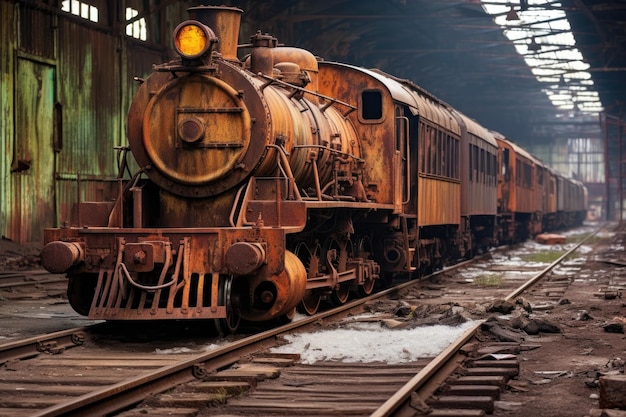This landscape-oriented image, likely a highly realistic AI rendering, captures a close-up and side view of a vintage steam locomotive in an abandoned, dilapidated train station. The rusted and dirty train, with its characteristic round yellow headlight and smokestack, boasts around eight cars extending into the distance. The train sits on the left-hand track, which, like the adjacent track, is broken and dotted with melting snow. The surrounding area is strewn with debris, wood, and patches of mud. The station itself shows signs of severe neglect, with broken windows in the ceiling, rusty green walls, and an overall air of desolation heightened by the absence of people.